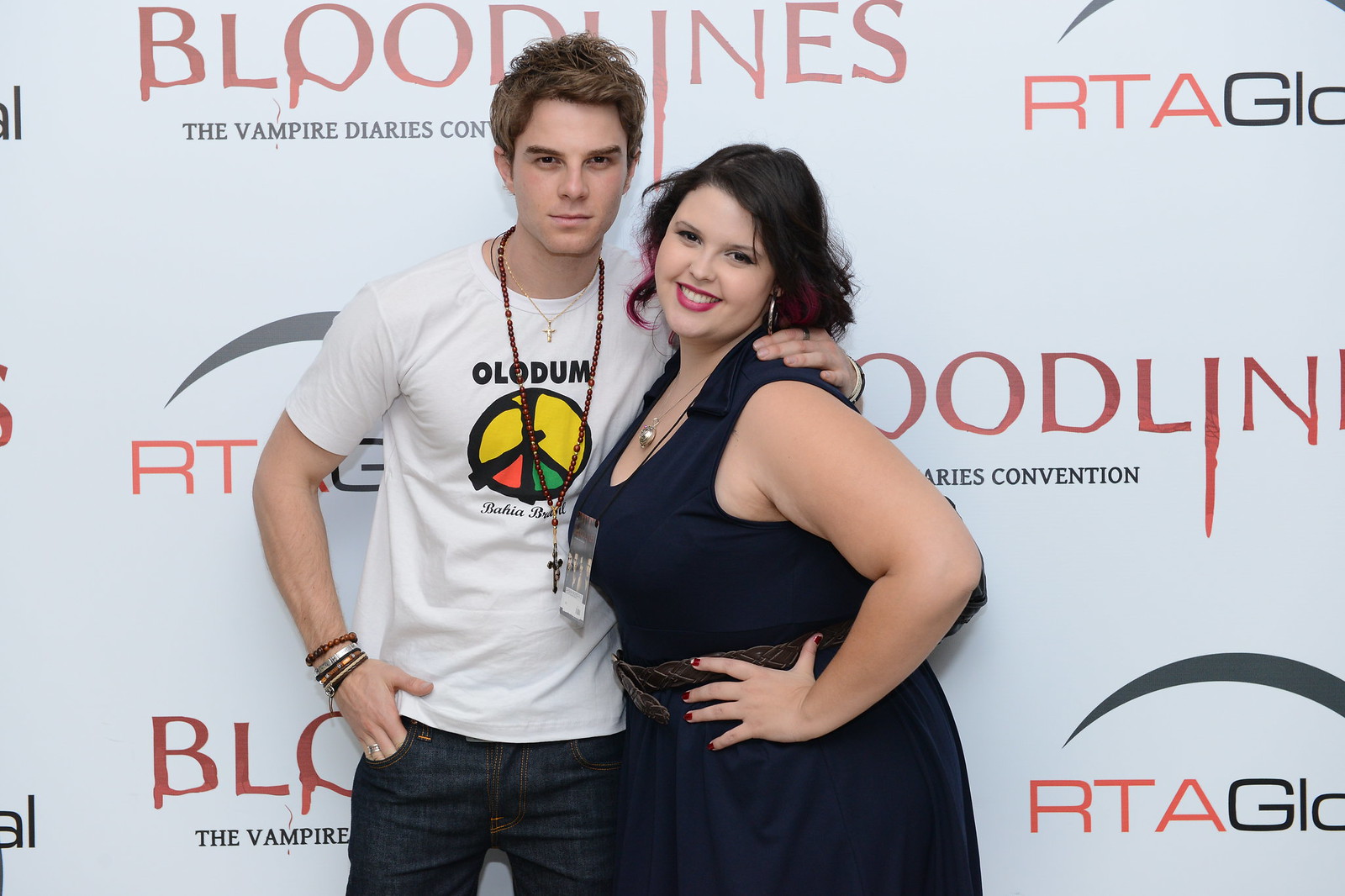In this detailed photograph taken at the Bloodlines: the Vampire Diaries Convention, two attendees are standing in front of a large promotional banner that spans the entire background. The man on the left is casually dressed in blue jeans and a white t-shirt with the words "Old Dumb" printed on it, featuring a peace sign logo. He accessorizes with a couple of long necklaces ending in crosses and several bracelets. His short brown hair tops off his laid-back look. He rests his left hand in his pocket while his right arm is draped around the shoulder of the woman beside him. The woman stands confidently in a blue dress, her sharp brown hair styled to shoulder length. She wears a lanyard around her neck, indicating her pass for the event, and has her hands placed firmly on her hips. Her red lipstick and beaming smile add an extra touch of vivacity. The background banner prominently features the event's title, "Bloodlines, the Vampire Diaries Convention," and an additional logo for "RTA Global." The overall scene suggests a lively atmosphere of fan engagement and celebrity interaction at this grand convention event.